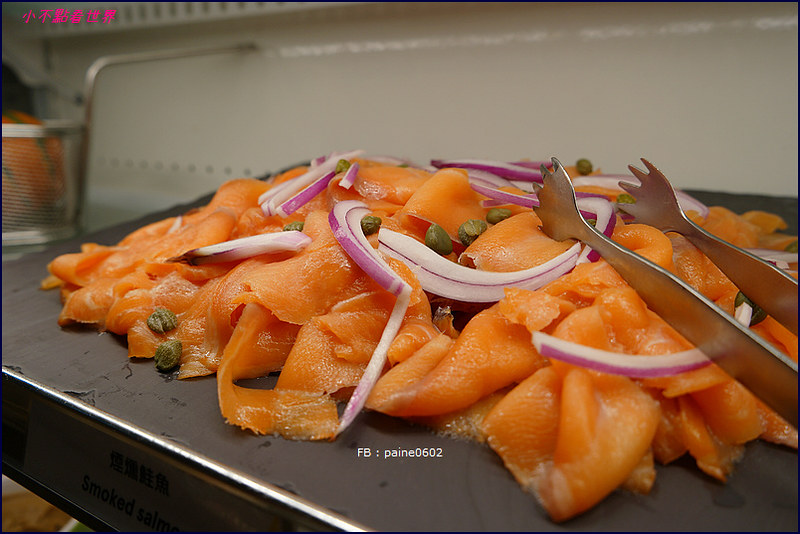This horizontal color photograph captures a plate of smoked salmon set on a gray metal scale, likely situated in a kitchen or supermarket setting. The salmon, thinly sliced and heaped in large piles, is adorned with slices of raw red onions and scattered capers. To the left of the plate, a metal basket filled with vegetables adds context to the environment. On the right side, a pair of stainless steel tongs rests, ready for serving. The image features Chinese characters in the upper left corner and the English text "FB: PAINE 0602" towards the bottom center, possibly indicating the photographer's handle. The scale prominently displays the label "smoked salmon" in English, with accompanying Asian script above it.